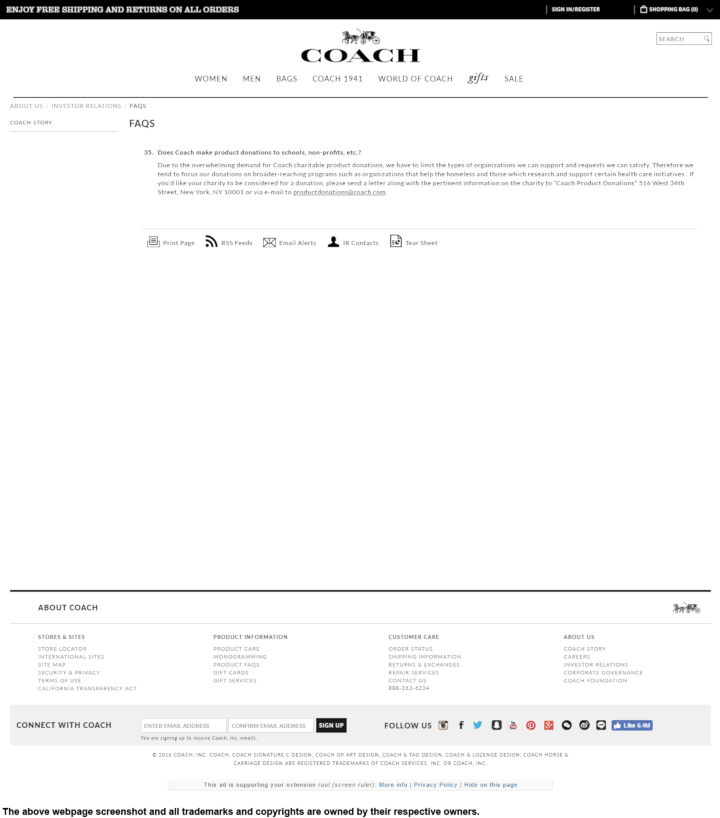This screenshot captures the homepage of the Coach website. Dominating the top of the page is the brand name "Coach" along with a distinctive logo featuring an image of what appears to be an Amish buggy pulled by two horses. The navigation bar directly beneath this logo includes clickable categories labeled: "Women," "Men," "Back," "Coach," "World of Coach," a cursive text (likely a stylized section name), and "Sale."

As you move down the page, the "Frequently Asked Questions" (FAQs) section is prominently displayed, having been clicked on to reveal a brief paragraph providing additional information. Below this section, five icons are arrayed horizontally, each representing different sections or functionalities of the website which users can navigate to.

Towards the bottom of the page, a solid black line extends horizontally across the width of the screen. The central portion of the homepage is notably plain, featuring minimal design or content. Finally, at the very bottom, the "About Coach" section offers additional information with four clickable links for further exploration.